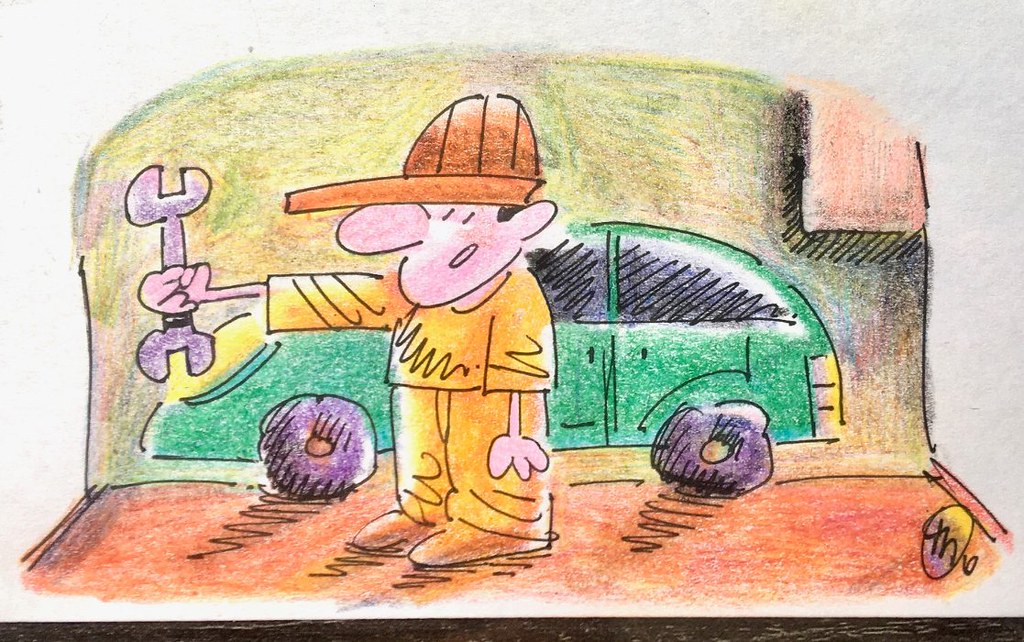In the center of a stark white background, a person is seated, prominently wearing an eye-catching orange hat. They are dressed in a stylish yellow shirt and bright orange shoes, adding vibrant splashes of color to the scene. One hand is extended outward, gripping a wrench. To the left of the individual is a vivid green car with black windows, positioned in such a way that both rubber tires are visible at the bottom left and bottom right of the image. An orange bar can be seen near the tires, and the bottom-right corner bears a distinct signature. Completing the setting, a red cabinet stands at the top right, adding another bold hue to the composition.